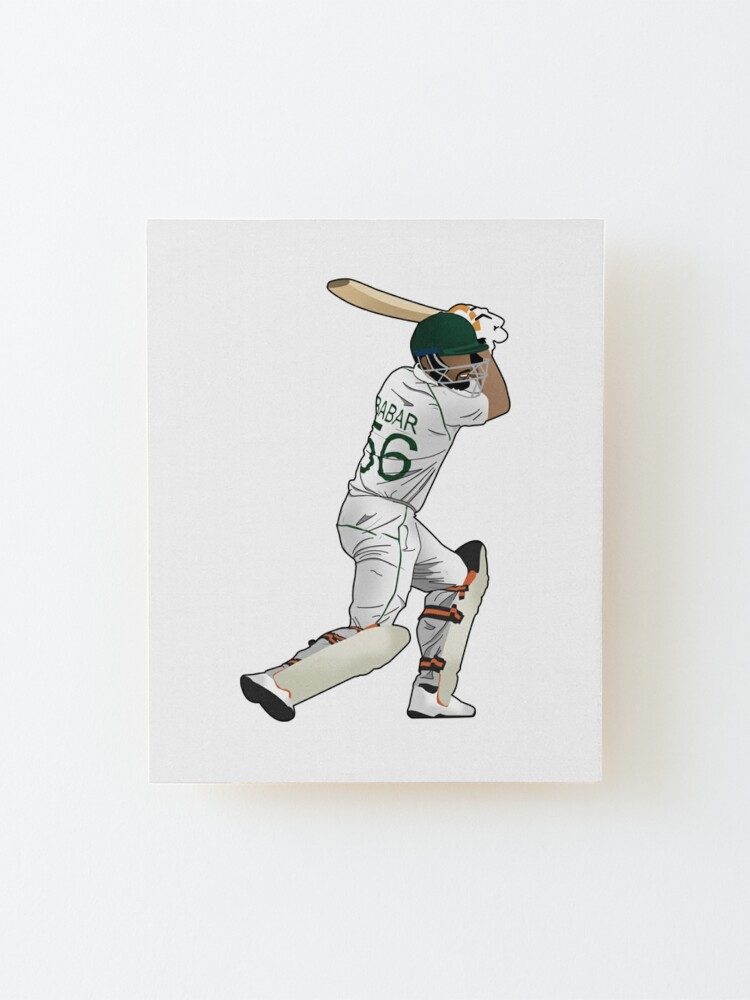This detailed illustration depicts a baseball player poised to swing his bat, capturing a moment of intense focus and readiness. The player, a dark-skinned male with a black beard, is adorned in a white uniform featuring green details, with his jersey prominently displaying the name "Rebar" and the number 56. His outfit also includes knee pads, reminiscent of those worn by hockey goalies, providing extra protection as he readies himself for the hit. He wears big gloves and sneakers, and his green helmet, equipped with a face protector, adds to his prepared stance. The man leans into his stance with his bat raised above his left shoulder, eyes locked onto the ball in keen anticipation. The sketch is set against a stark white background, making it a perfect decorative piece for any baseball enthusiast's wall.